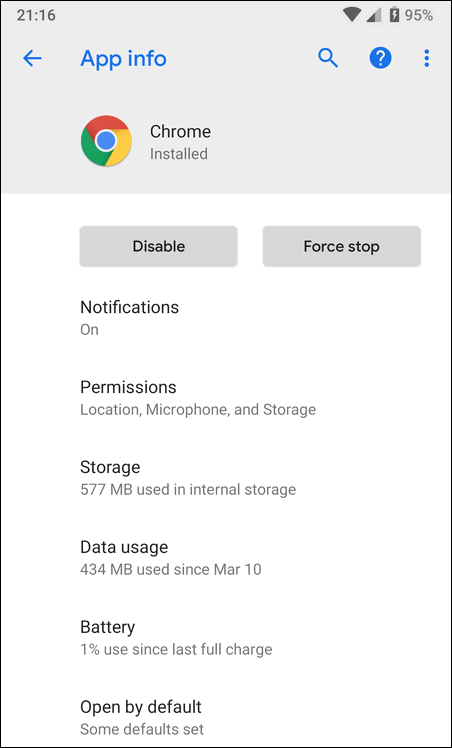The image is a detailed screenshot taken from an Android phone, specifically showing the information section of the Chrome app. At the top-left corner of the screenshot, the time is displayed as 21:16 (9:16 PM). On the top-right corner, several status icons are visible, including the Wi-Fi icon, the cellular data icon, the charging battery icon, and the battery percentage, which is at 95%.

Directly below this top bar, the heading "App Info" is centered. Beneath this heading, there is a line of text stating "Chrome installed," indicating that the Chrome app is installed on the device. Directly beneath this text, on the left side, is a button labeled "Disable," and to the right of it is another button labeled "Force Stop."

The following sections provide more information about the app's settings and usage:
- **Notifications:** Listed as "On."
- **Permissions:** Includes Location, Microphone, and Storage permissions.
- **Storage:** Shows that the Chrome app is using 577 MB of internal storage.
- **Data Usage:** Indicates that the app has used 434 MB (although the time frame is not specified).
- **Battery Usage:** Displays that the app is currently consuming 1% of the battery.
- **Open by Default:** The status of this setting is not specified.

Overall, the screenshot comprehensively details the current state of the Chrome app as seen through the Android settings menu.